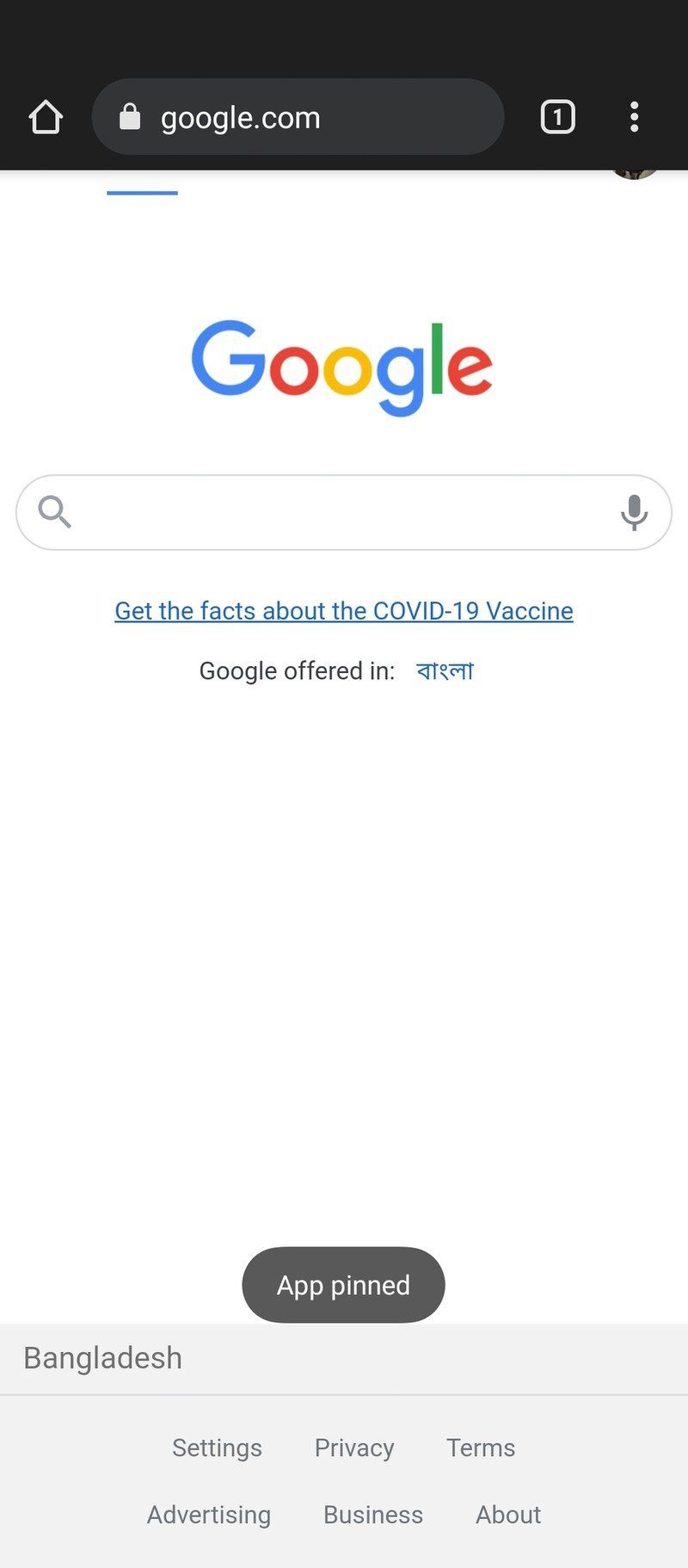This screenshot captures a detailed view of the Google homepage. The image is vertically oriented, with a greater height than width. 

At the very top, there's a two-inch black border. About one inch from the top, you'll find a white home icon with a black center and white border. Beneath this, a search bar extends roughly halfway across the screen. Within the search bar, a white lock icon and the text "Google.com" are displayed in white. To the right of this, there’s a white-outlined box with a black interior featuring a white numeral "1", followed by two white dots.

Directly underneath the lock icon and white border runs a thin blue line, approximately one inch long. Centered about two inches below the black border is the iconic Google logo, spelled with a blue "G", red "O", yellow "O", blue "G", green "L", and red "E". Below the logo, a prominent search bar spans the width of the screen, containing a microphone icon on the right and a search icon on the left.

Beneath this search bar, in blue text, an underlined link reads: "Get the facts about COVID-19 vaccine." Below this link, in black text, it says: "Google offered in", followed by what appears to be Chinese characters in blue.

Approximately three inches down, a centered gray tab contains white text that reads: "App pinned." The background below this section transitions to light blue. On the left side, the word "Bangladesh" is written in black and underlined. In the center and below this, the words "Privacy" and "Business" are written, with "Settings" and "Advertising" to the left, and "Terms" followed by "About" to the right.